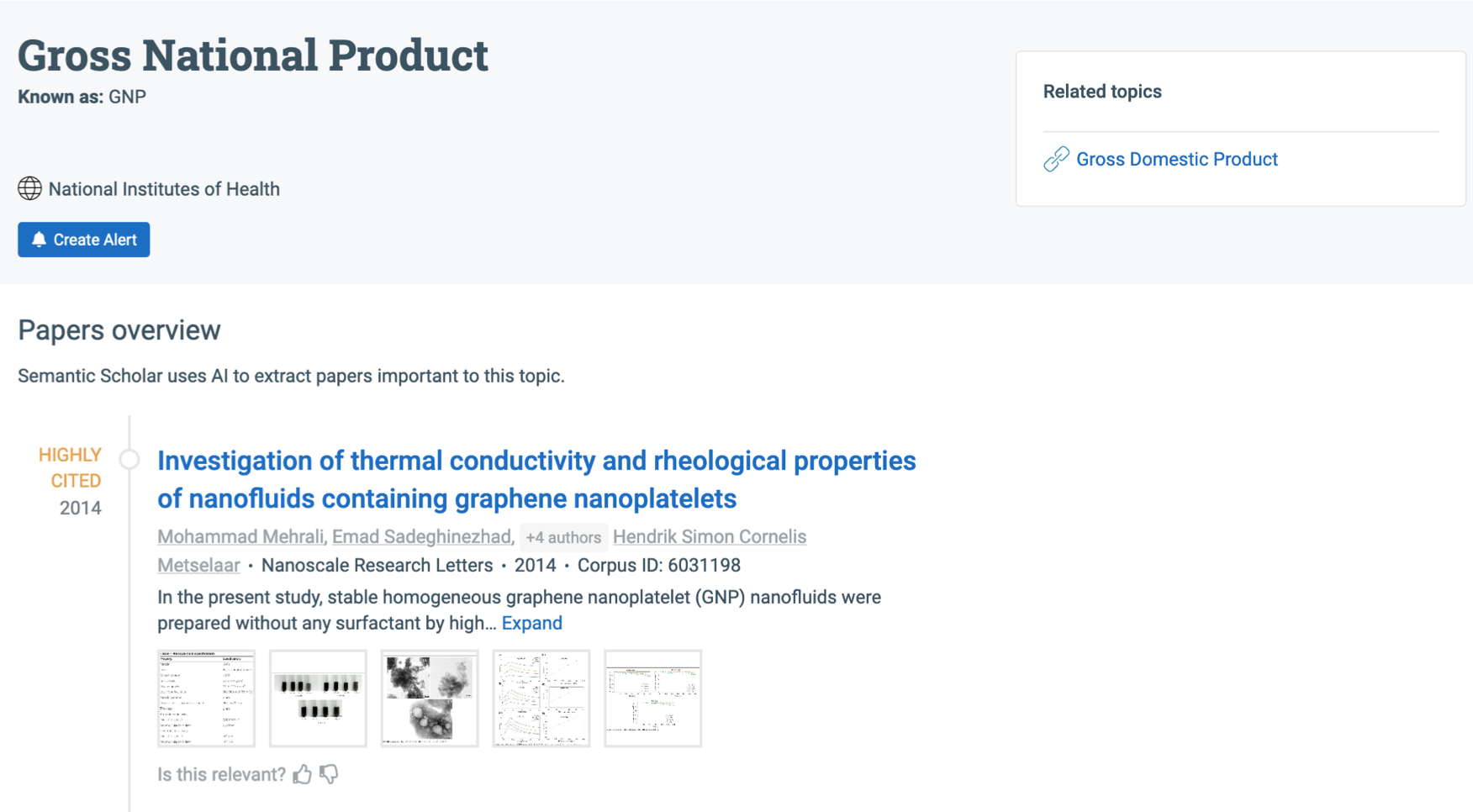This image, captured from a computer's website, presents various elements associated with economic and academic content. At the top of the image, there is a faint gray rectangle wherein the term "Gross National Product" is prominently displayed in black print on the top left. Directly beneath it, "GNP" is specified as an abbreviation. 

Below this section, a globe icon is visible alongside the text "National Institute of Health." Adjacent to this, a blue rectangle with white text reads "Create Alert," accompanied by a bell icon.

To the far right edge of the image, there is a white rectangle containing the text "Related Topics" in black print.

At the bottom of the image, the term "Gross Domestic Product" is displayed, complete with an infinity sign next to it. The entire lower section of the background is white, featuring a heading titled "Pages Overview." Underneath this heading, in smaller print, is the explanation: "Semantic Scholar uses AI to extract papers important to this topic." Following that, in blue print, is the description of a research paper titled "Investigation of Thermal Conductivity and Rheological Properties of Nanofluids Containing Graphene Nanoplatelets."

Additionally, five small diagrams are arranged at the bottom of the image, presumably related to the research paper mentioned.